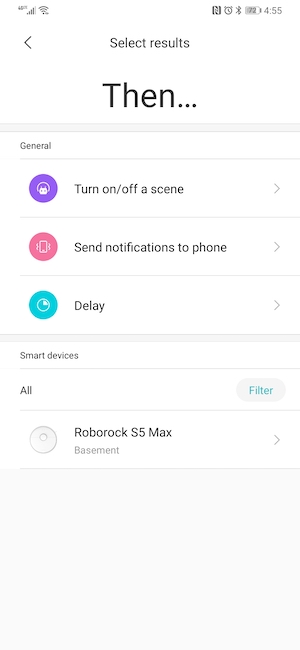This image depicts a mobile device screen showcasing a user interface with several interactive elements. At the very top, the screen displays common device information such as the battery life at 72% and the current time, 4:55 PM, with icons positioned on both the left and right of the status bar. The primary section of the screen prominently features the text "Select results" followed by "then..." in large black letters, accompanied by a left-pointing arrow icon.

Below this main header, the interface is divided into distinct functional areas. First, there is a general section displaying a purple button, accented with a bug icon, labeled "Turn on/off a scene." Following this is a pink button, adorned with an icon of a vibrating phone, labeled "Send notifications to phone." 

Continuing downward, there is an area highlighting a teal icon with a clock symbol in the center, labeled "Delay." Each of these options includes a right-pointing arrow at the end of their respective lines, indicating the potential for further action or navigation.

At the bottom portion of the screen, under the section titled "Smart devices," there is a subsection labeled "All" with an adjacent filter button for customization. Below this, the display lists a device named "Robo Rock S5 Max Basement," indicating a connected smart device available for user interaction.